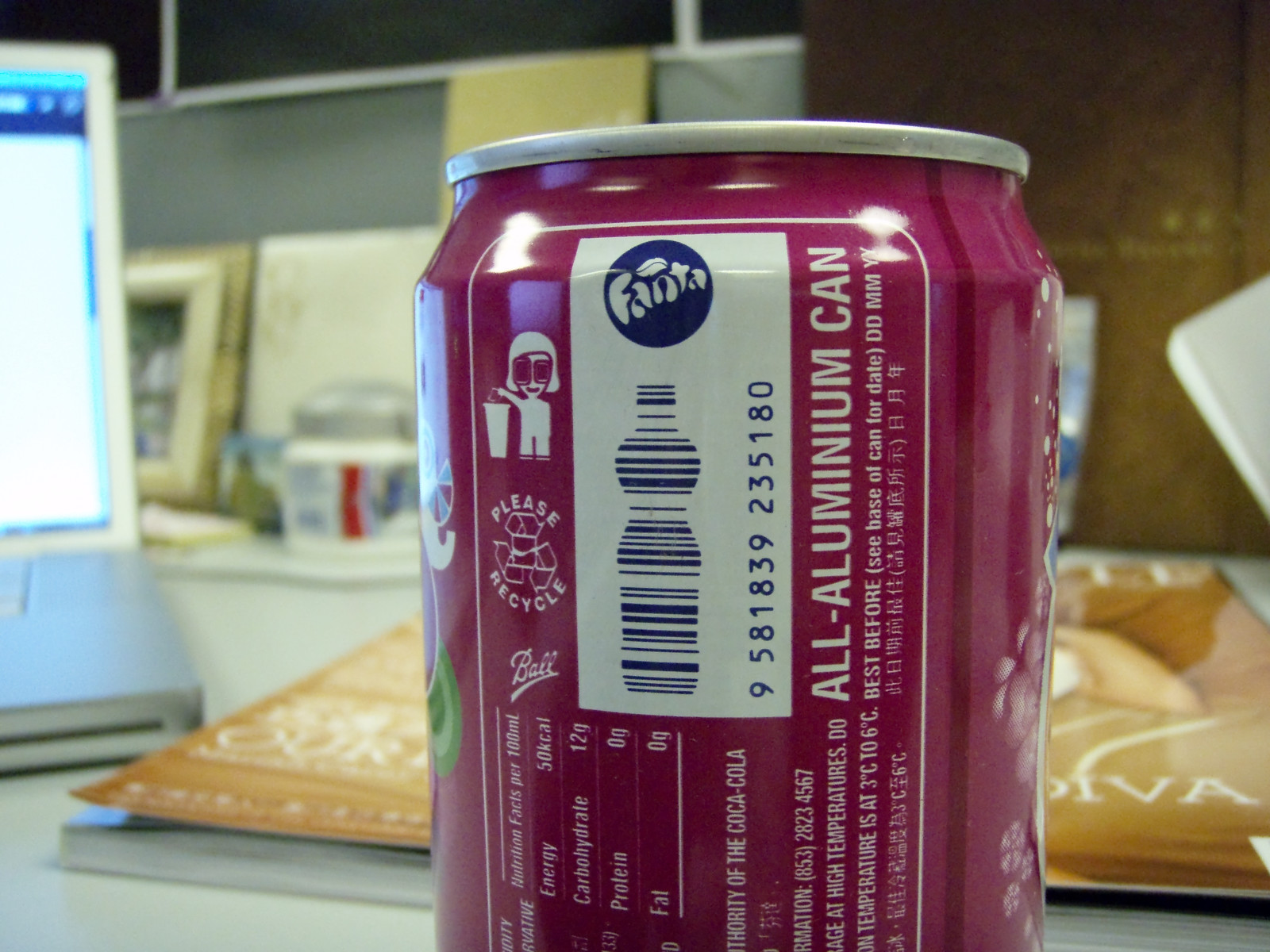A vivid scene depicts a cherry-flavored Fanta soda can prominently displayed on a tabletop. The can is adorned with vibrant red and white branding, indicative of its fruity contents. Positioned behind the can are two pastries, each protected by crinkled plastic bags; one pastry is clearly discernible while the other remains ambiguous in content. The right side of the can features a barcode and associated numeric sequence. This tableau is situated in a cozy setting that includes a double wooden door in the backdrop, enhancing the homely atmosphere.